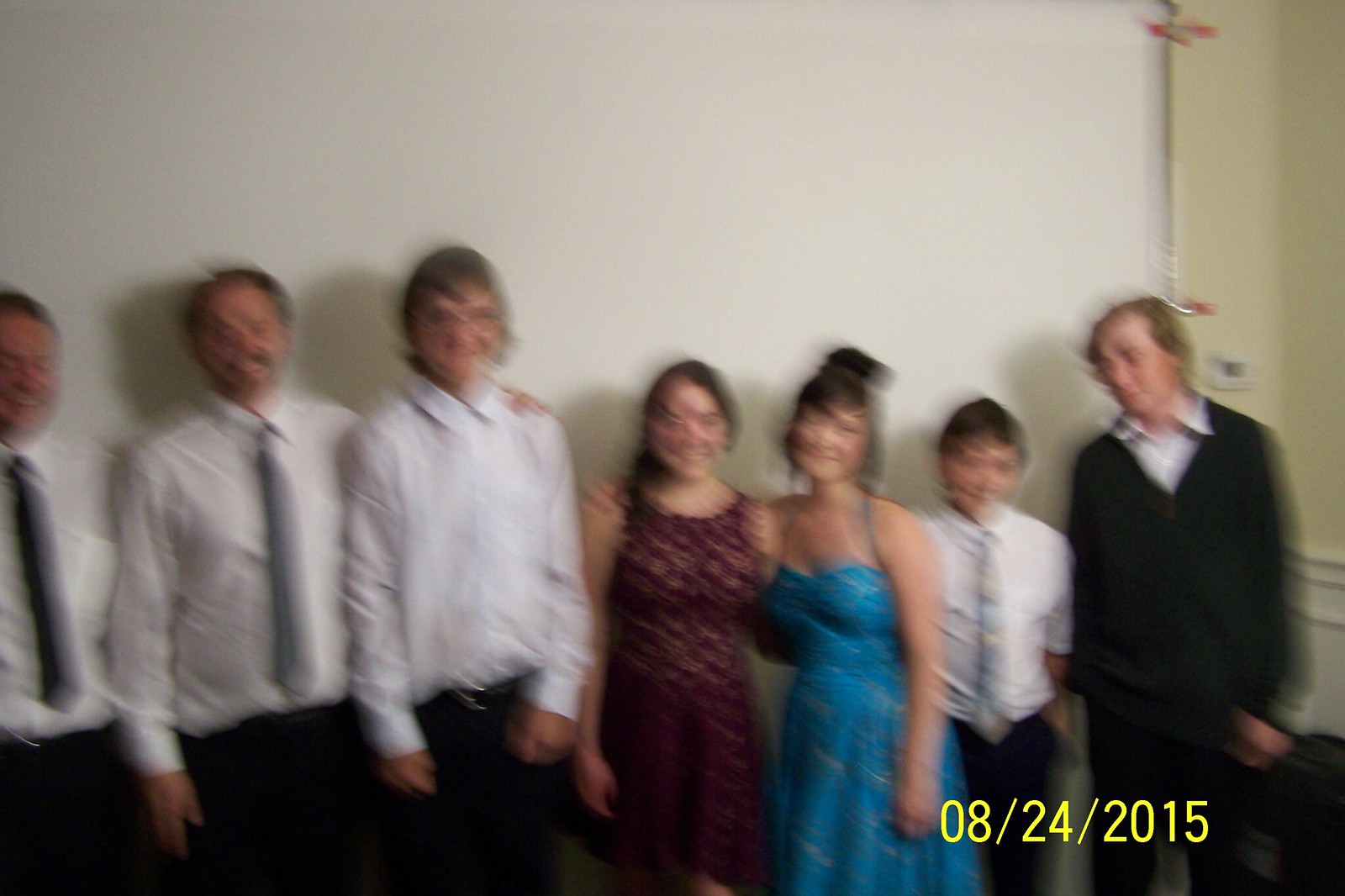This photograph, taken on August 24, 2015, depicts a group of seven individuals standing against the corner where two walls meet. From right to left, the first three are males, all dressed in white shirts and black pants. The first two appear to be older men, distinguished by their white ties, while the third is a younger male, similarly attired but without a tie. Following them is a woman in a burgundy dress, then another woman wearing a teal dress. Next stands a young boy, wearing a white shirt, black pants, and a tie. The last person is a teenager dressed in a white shirt and a black sweater. The image appears noticeably blurry, obscuring finer details. A timestamp in yellow, located in the bottom left corner, reads "08-24-2015."